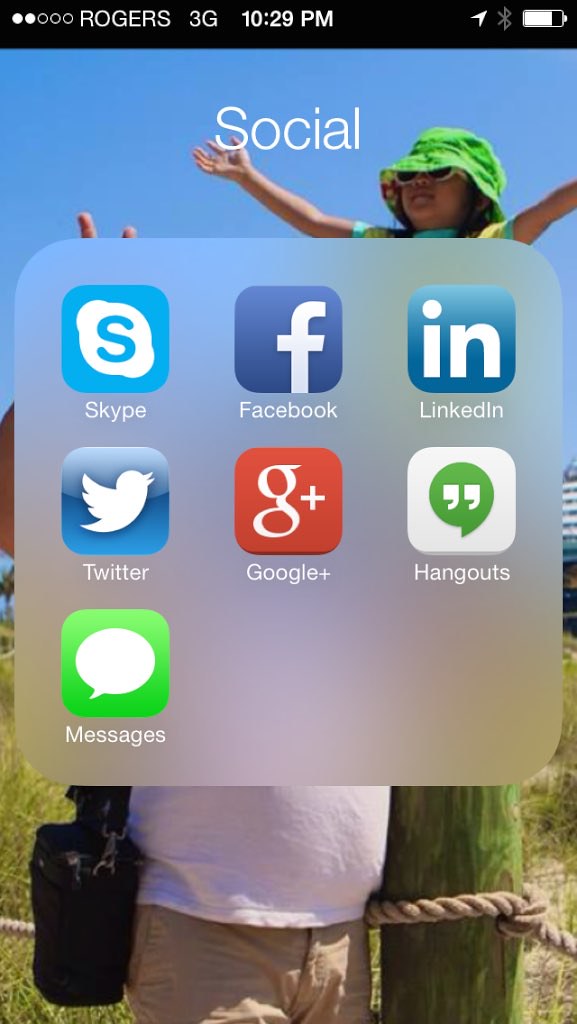The screenshot showcases the home screen of a smartphone, featuring various social media app icons against a black border. The status bar at the top indicates a 3G connection, the time as 10:29 PM, and a battery level at approximately 75%. Two out of five indicator dots at the bottom are white, while the rest are black.

Central to the image, there is a photograph of a sunny outdoor scene. A little girl, sitting atop a wooden post, poses with her arms outstretched as if to give a huge hug. She has two thick, braided pigtails. Beside her stands a man wearing a white t-shirt, a khaki-colored bottom, possibly shorts or pants, and a camera bag slung across his body. He is captured making a peace sign with his hand, wearing sunglasses and a yellow sailor hat.

In the background, there are patches of grass, sand, and weeds suggesting the location is near a beach.

The forefront of the screen displays a collection of social media app icons including Skype, Facebook, LinkedIn, Twitter, Google Plus, Hangouts, and Messages. Above these icons, there is the word "Social" denoting the folder's purpose.